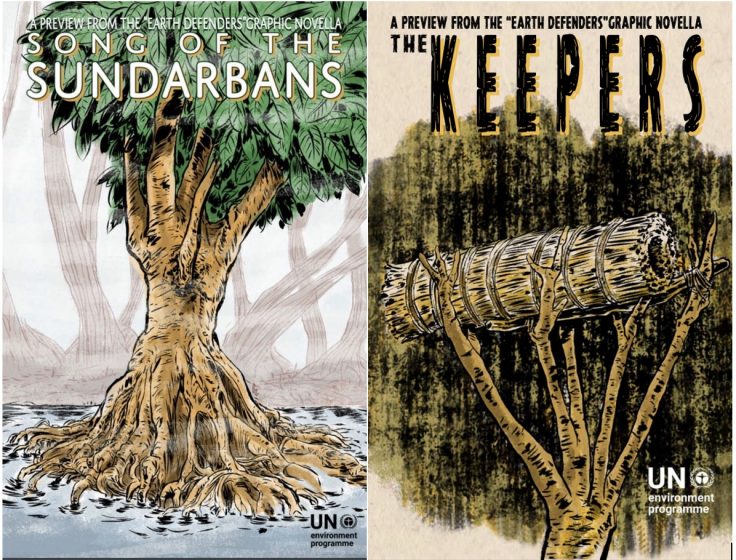The image showcases two distinct posters, each featuring a preview from the Earth Defenders graphic novellas, presented by the UN Environment Program, as indicated by their logos in the lower right corners. 

The left poster illustrates a unique tree with exposed roots above water, light brown in color with an abundance of large green leaves. The title at the top reads: "A preview from the Earth Defenders graphic novella, Song of the Sundarbans," capturing a vibrant and lush scenery.

Contrastingly, the right poster adopts a dark and somber yellow and black palette. It depicts a barren tree with dry, leafless branches, holding aloft a bundled haystack at the top. The top of this poster states: "A preview from the Earth Defenders graphic novella, The Keepers," emphasizing a more desolate environment.